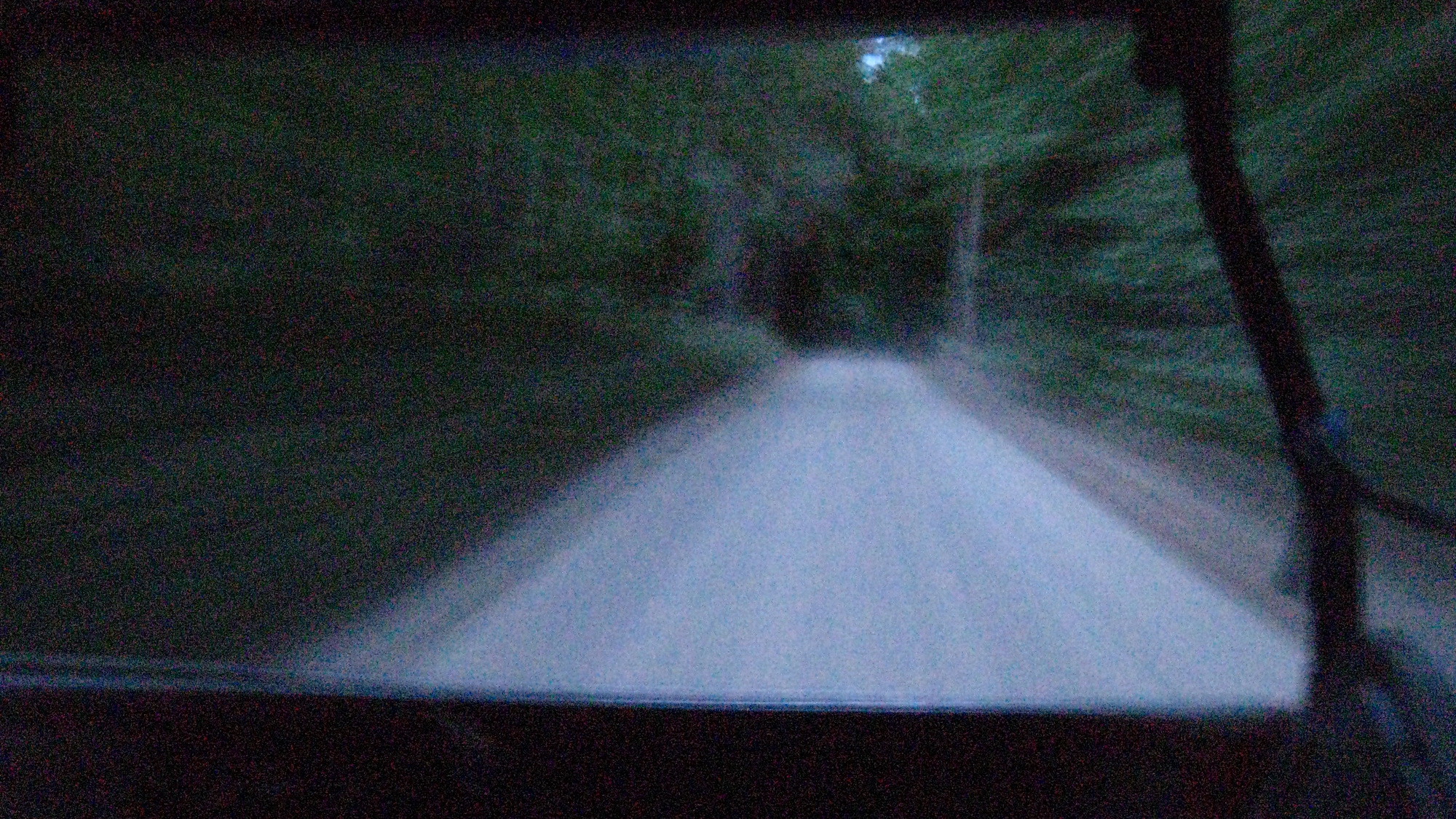The photo captures a dynamic, first-person perspective from a moving vehicle, potentially a windowless golf cart or jeep, racing down a gravel driveway lined with bricks and dirt planters. The surrounding environment is a dense, lush forest with numerous types of trees featuring long, thin brown trunks and abundant leaf coverage, creating a tunnel-like effect. The motion of the vehicle adds a sense of speed, rendering the image somewhat blurry. A small patch of blue sky is faintly visible at the far end of the driveway, adding a touch of light to the otherwise shaded scene.